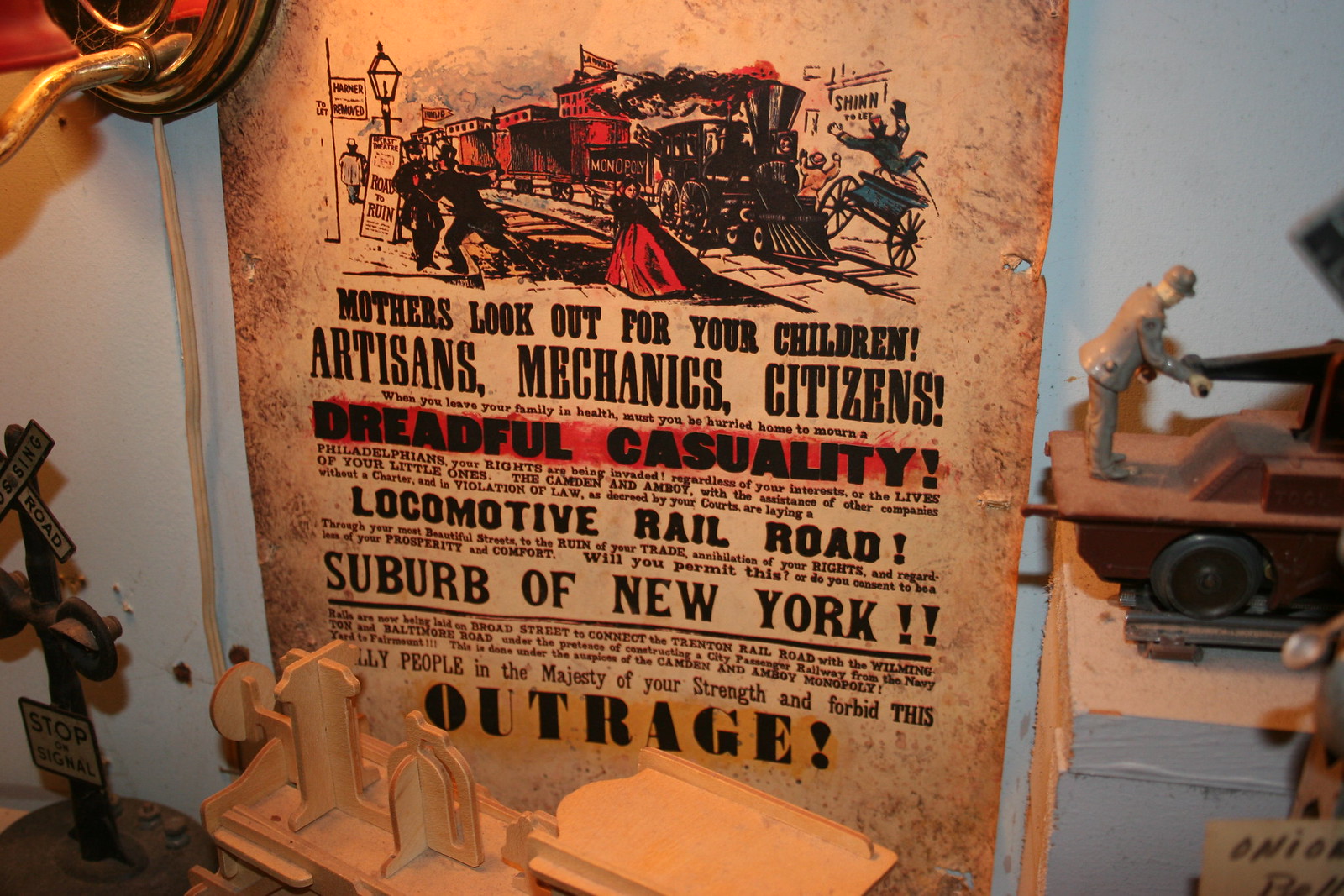The image displays a detailed, historical poster prominently set up on a table surrounded by various figurines and toys. The poster features a vivid drawing of a locomotive with red cars and a black engine depicted colliding with a horse-drawn carriage, causing chaos among the people. The train has the word "Monopoly" labeled on its side, symbolizing the aggressive encroachment it represents. Below the illustration, the poster delivers an urgent message: "Mothers, look out for your children. Artisans, mechanics, citizens, when you leave your family in health, must you hurry home to mourn a dreadful casualty? Philadelphians, your rights are being invaded. Regardless of your interests or the lives of your little ones, the Camden and Amboy, with the assistance of other companies without a charter and in violation of law as decreed by your courts, are laying a locomotive railroad through your most beautiful streets to the ruin of your trade, annihilation of your rights, and regardless of your prosperity and comfort. Will you permit this, or do you consent to be a suburb of New York?" The poster concludes with the word "OUTRAGE" in bold letters at the bottom. Surrounding the poster are miniature model toys, including a railroad car with a figurine pumping a handcar, a model car, and a railroad crossing sign, all placed against a white wall in the background. The display combines historical protest with playful diorama elements to create a visually engaging scene.